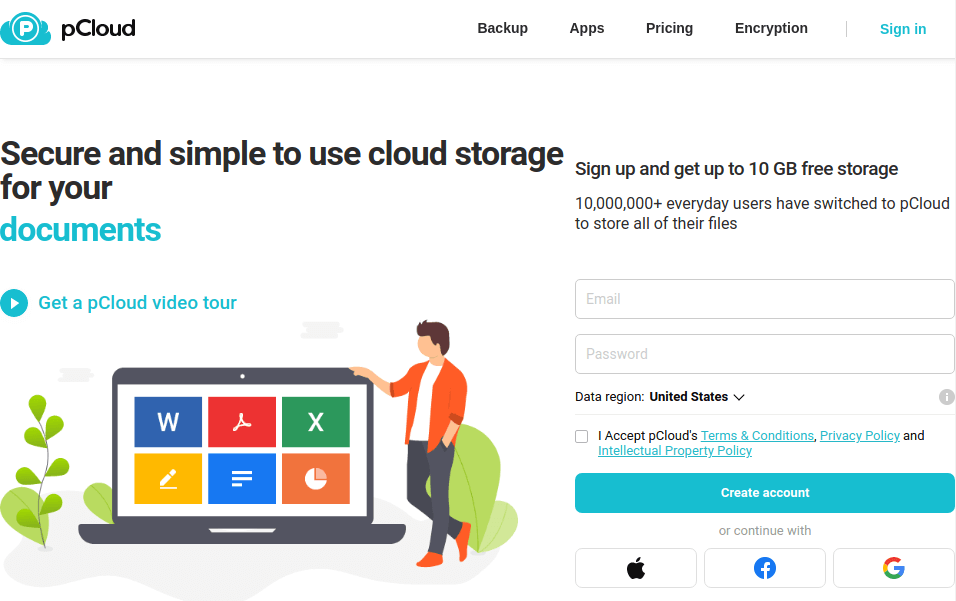The screenshot captures the homepage of the pCloud website. On the left-hand side, there is a prominent cloud icon with a circle around it, bearing a bold white letter "P". 

In the middle-right section of the page, the menu includes options such as "Backup," "Apps," "Pricing," "Encryption," followed by a vertical separator line, then "Sign In", which is highlighted in sky blue. Below this line, an informative text titled "Secure and simple to use cloud storage for your documents" appears, with the word "Documents" highlighted in sky blue.

Beneath this, there is a play button enclosed in a sky-blue circle featuring a right-pointing arrow, accompanied by the text "Get a pCloud video tour," also highlighted in sky blue.

Lower on the page, an image depicts a laptop with cartoon-like clip art of a person placing their hand on top of it. The cartoon character is almost the same height as the laptop. 

To the right, near the top, there is a sign-up prompt: "Sign up and get up to 10 GB free storage," followed by another message stating: "10,000,000+ everyday users have switched to pCloud to store all their files."

Below this, there are fields for "Email" and "Password", a drop-down menu for "Data Region" defaulting to "United States," a checkbox for accepting pCloud's terms and conditions, and a button labeled "Create Account". At the bottom, three social media icons are displayed.